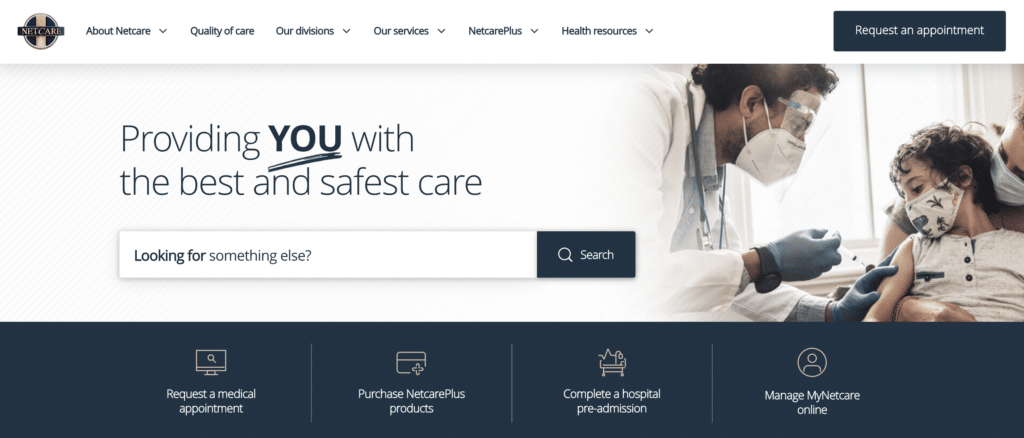This is a screenshot of the Net Care website. The top header bar features six tabs: About Net Care, Quality of Care, Our Divisions, Our Services, Net Care Plus, and Health Resources. On the extreme right of the header is a "Request an Appointment" button. The main image depicts a healthcare practitioner carefully administering a vaccine to a young child. The practitioner is equipped with a face mask, a protective visor, blue latex gloves, a stethoscope around their neck, and a white lab coat. The child, who is also wearing a face mask and a sleeveless shirt, is held by a parent wearing a white face mask. The setting appears to be a well-lit room with a window in the background. Overlaying the photo is a blue text banner that reads: "Providing you with the best and safest care." Below this text is a search bar for easy navigation.